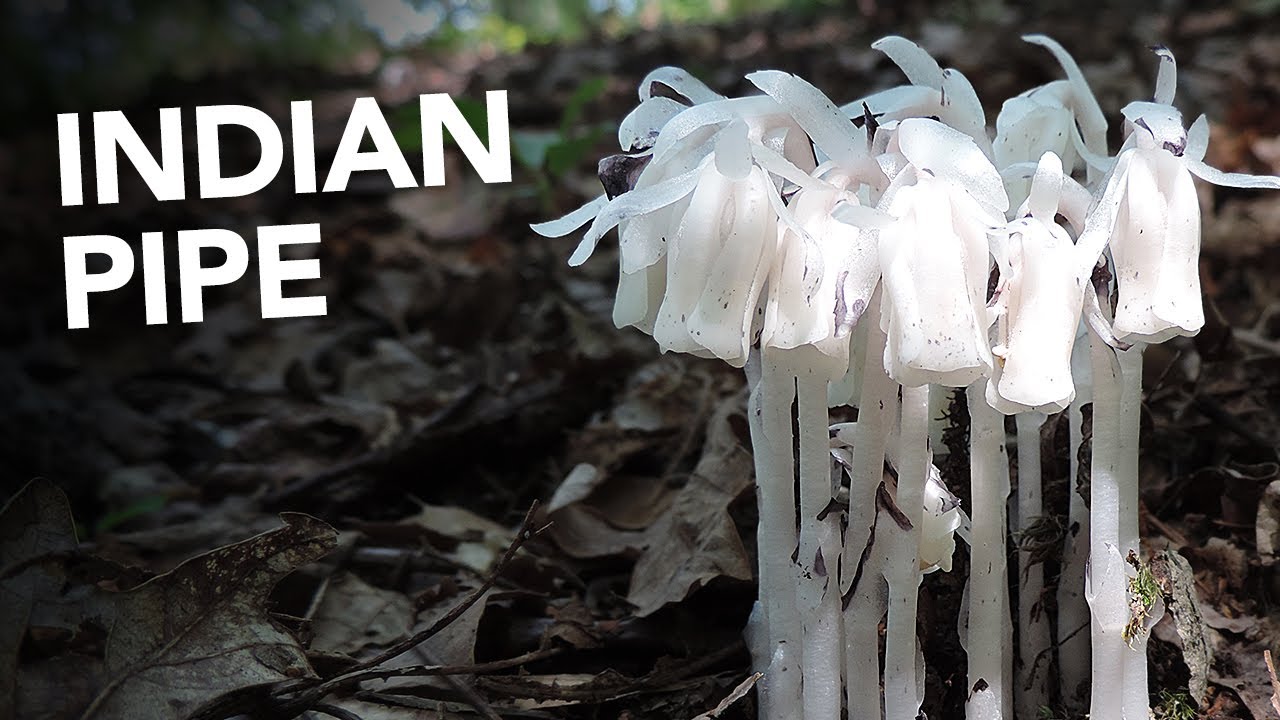The landscape-oriented photograph prominently features an unusual plant called Indian pipe, indicated by bold, white, all-capital text in the upper right corner of the image. On the right side of the photo, the focus is on strikingly white, slender stalks emerging from a thick bed of dark, dead leaves scattered across the ground. These stalks transition into delicate, drooping white flowers that resemble wilted tulips, each adorned with subtle purple specks. In the far background, some blades of grass can be seen protruding from the leaf litter, adding an additional layer of texture to the scene. The overall composition draws attention to the intriguing and ghostly appearance of the Indian pipe plant, standing out against its somber backdrop.